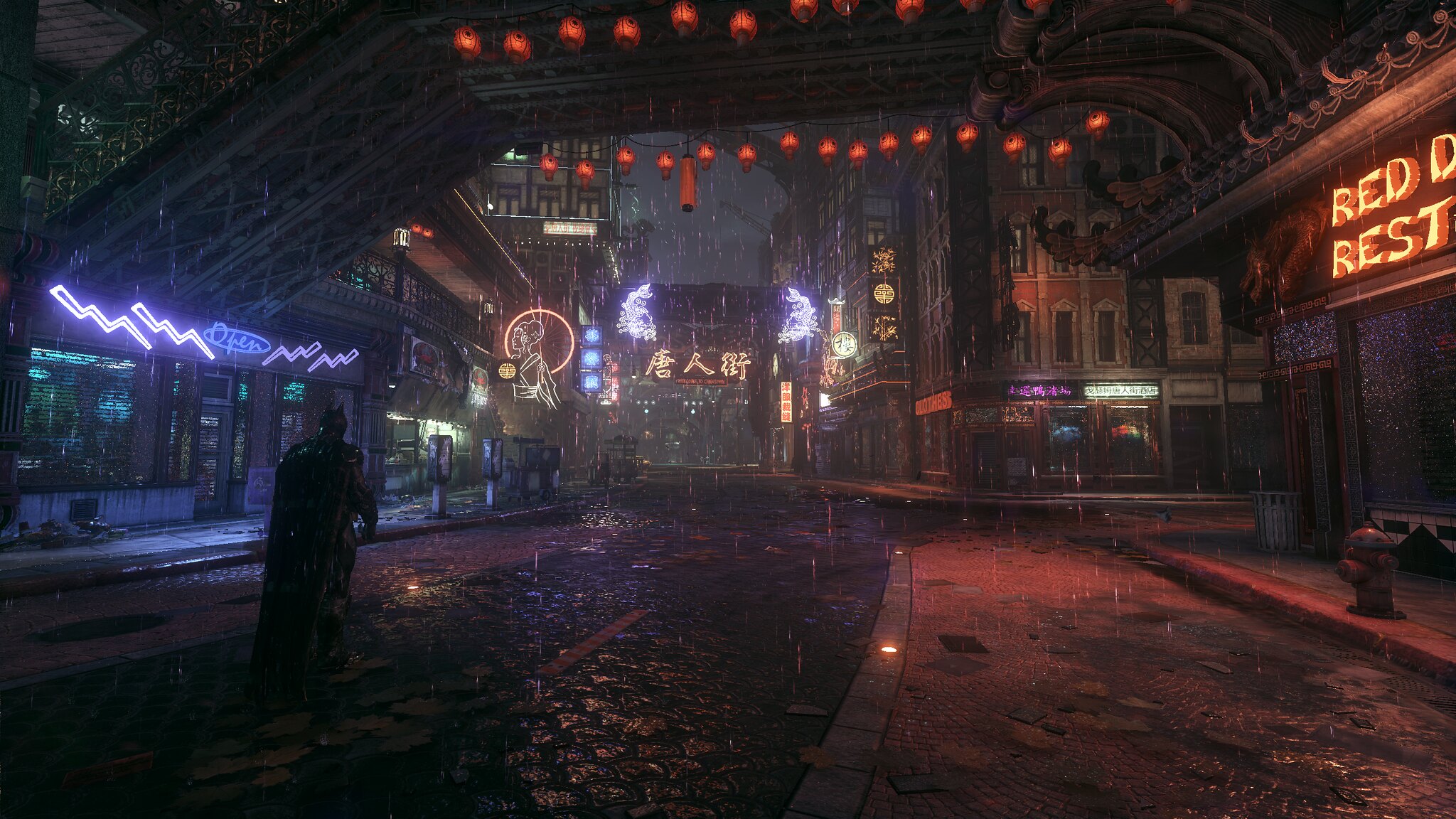In this detailed image, we see a vividly illuminated scene, probably from a movie or video game, set in a bustling Asian city, possibly Chinatown, at night. The scene unfolds under a downpour, with raindrops visible on the stone-paved streets, which reflect various colored lights. Despite the brightness of the numerous neon lights, the street itself is devoid of people, giving it a desolate yet vibrant atmosphere. On the right side of the street, a brightly lit sign reads what appears to be "Red Dragon Restaurant" with its distinct neon glow. Contrastingly, the signs on the left are in Chinese and include traditional red lanterns that hang above, further enhancing the cultural ambiance.

At the heart of the scene, a lone figure enclosed in black – broad-shouldered, with a cape and ears reminiscent of Batman – walks away from the viewer, adding a mysterious element to the setting. His silhouette is highlighted by the reflective red and purple neon lights around, casting an eerie glow over the wet street. The background buildings, crafted from red brick, are adorned with several other signs, one notably lit with purple kanji, contributing to the overall dynamic and immersive street view. The scene captures the essence of a cinematic detective noir combined with the vibrant essence of an urban Asian nightscape.